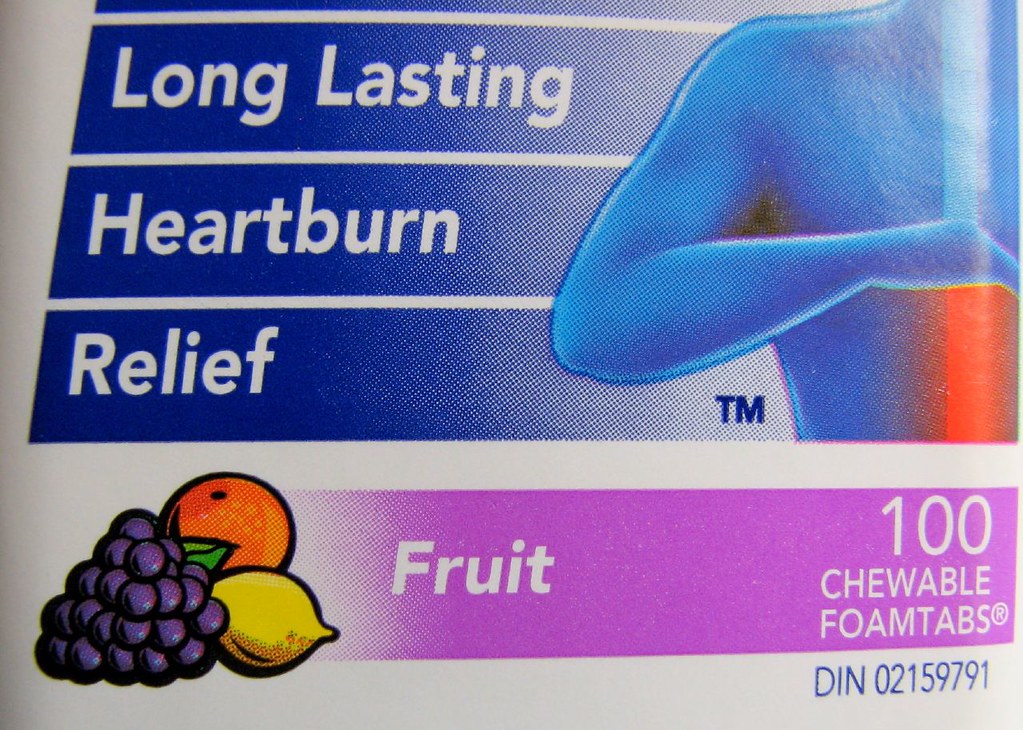This photograph features packaging for a medication product specifically designed for long-lasting heartburn relief. The packaging prominently displays text against blue strips, with bold white font broken into three sections reading "Long-Lasting Heartburn Relief." 

To the right of this text, there's a graphic of a blue human figure with a bent elbow, highlighting a red area towards the lower part of the body, likely indicating the region where heartburn occurs. 

On the left side of the packaging, a cluster of fruits is depicted, including purple grapes, an orange, and a yellow lemon, next to a purple strip. The strip bears white text stating "Fruit" on one side and "100 Chewable Foam Tabs" on the other. Below this, in blue font, is the drug identification number, "DIN 021-59791." The photograph also captures a subtle light reflection across the image, adding a touch of realism.